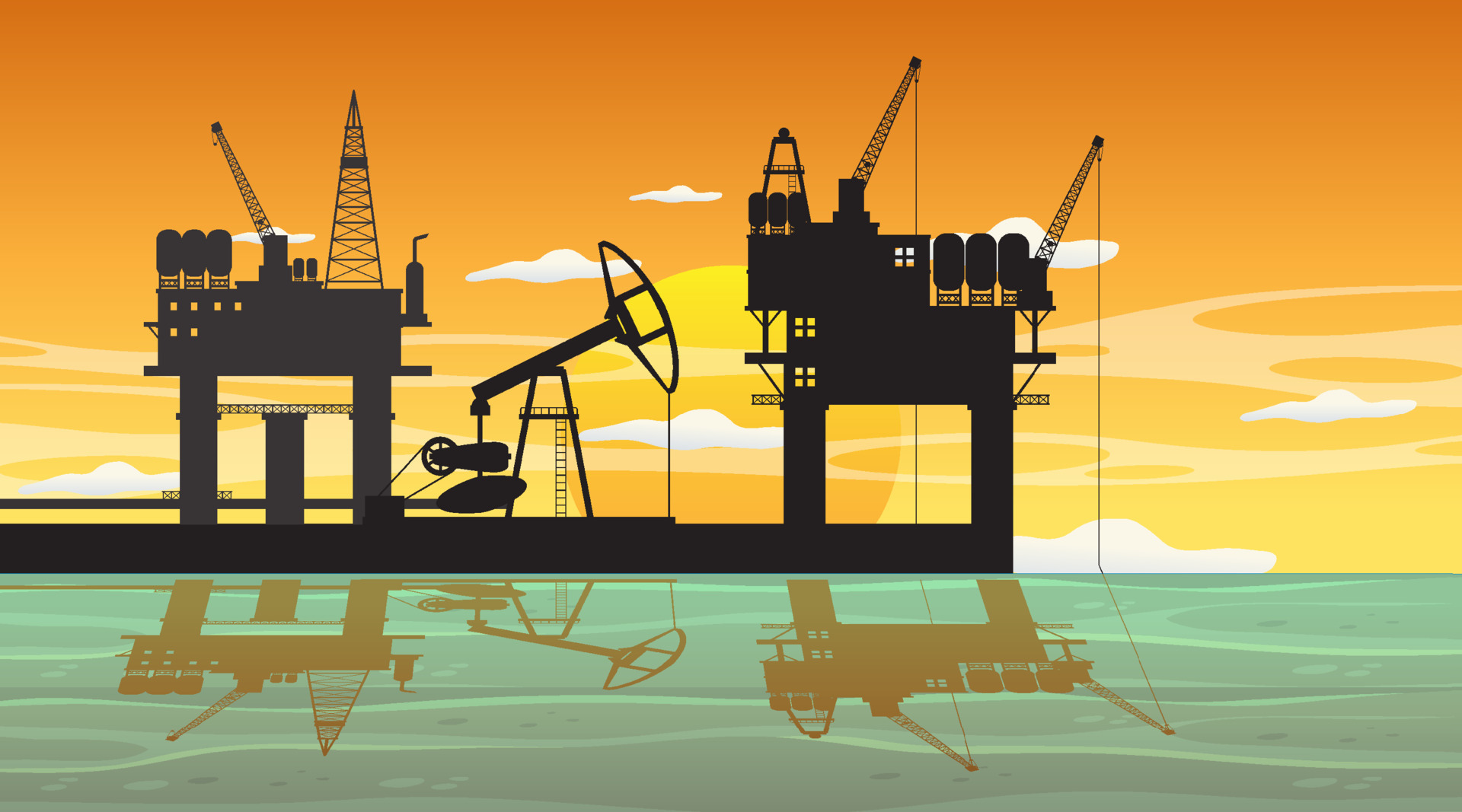This detailed cartoon image features a modern, minimalist depiction of an oil drilling rig silhouetted against a striking background of an orange and yellow sky, indicative of either sunrise or sunset. The sky, adorned with a few wispy clouds, transitions into darker hues at the top. The central focus of the image is the oil rig, composed of three main parts: two table-style drilling platforms on either side and a central hammer mechanism for drilling. Each element of the rig is rendered in black, contributing to its professional and defined appearance. The rig stands above a body of water, which is illustrated in a paler blue, capturing the rig's precise silhouette in its reflective surface. The setting sun adds a golden glow, enhancing the reflection and shadows of the structures in the water below. This artistic rendering, likely computer-aided, vividly captures the scene with clear outlines and intricate details, giving it a realistic yet stylized look, without any text to distract from the visual elements.